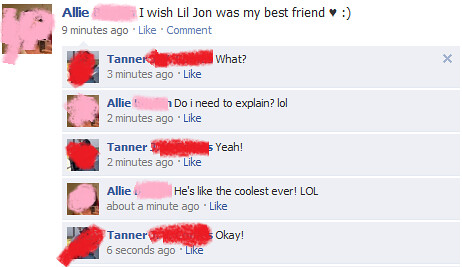This image is a detailed screenshot of a Facebook post's comment section. The post, made by a user named Ally nine minutes ago, reads, "I wish Lil Jon was my best friend" accompanied by a black heart emoji and a smiley face. The profile pictures and last names of the participants are obscured by a red and pink brushstroke effect. The background colors of the screenshot include hues of white, blue, pink, tan, black, dark blue, and gray. Below Ally's original post, Tanner comments "What?" three minutes ago. Ally responds, "Do I need to explain? LOL," two minutes ago. Tanner replies, "Yeah," also two minutes ago. Ally then elaborates, "He is like the coolest ever. LOL," about a minute ago, followed by Tanner’s final reply, "OK," made six seconds ago. Throughout the thread, the "like" and "comment" options are visible alongside each interaction. The screenshot is centrally positioned in the image with no other objects or elements worth noting. The setting distinctly resembles a social media app, likely Facebook.